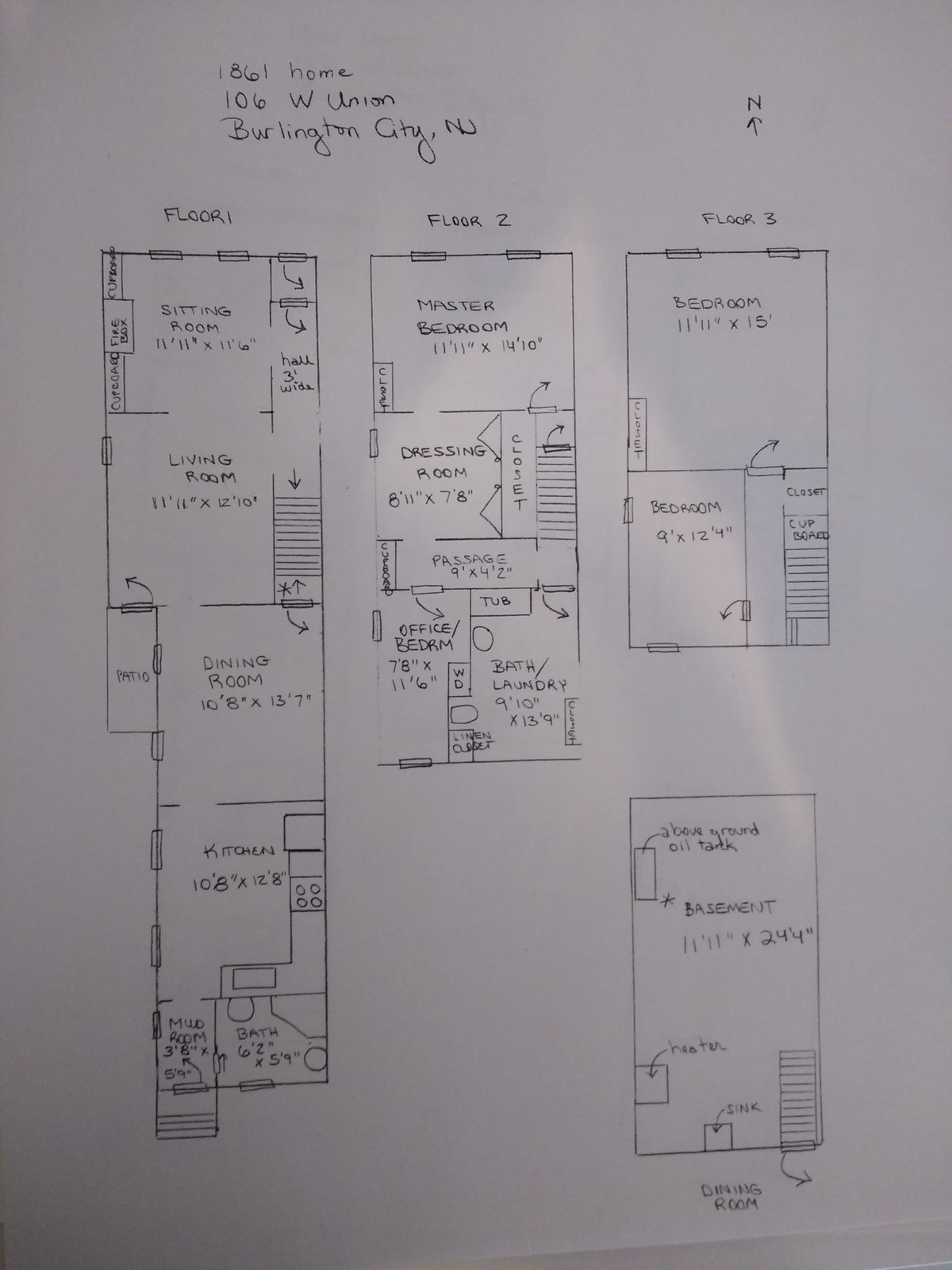Caption: 

A meticulously hand-drawn set of floor plans for a historical house at 106 West Union, Burlington City, New Jersey, dated 1861. Crafted with precision using a straight edge and pen on a white sheet of paper, the plans feature a north arrow in the top right corner for orientation. 

The upper left corner is labeled with three lines of text: "1861 Home," "106 West Union," and "Burlington City, New Jersey."

The floor plans are divided into four sections: "Floor 1" on the left, "Floor 2" in the middle, "Floor 3" on the right, and a "Basement" in the bottom right corner. Dimension details are provided for each room, and staircases are represented by striped lines. 

Floor 1 includes areas designated as a sitting room, living room, dining room, kitchen, bathroom, and possibly another room that is difficult to decipher. 

Floor 2 features a master bedroom, dressing room, an undecipherable room (potentially labeled as "painting"), an office/bedroom, and a bath/laundry room.

Floor 3 specifies room dimensions more precisely, with a bedroom measuring 11 feet 11 inches by 15 feet and another bedroom measuring 9 feet by 12 feet 4 inches.

The layout also details the stair and door placements, indicating the direction in which doors open. Windows are depicted as rectangles that overlap the walls' outer borders, enhancing the comprehensive nature of the plans. 

Overall, these hand-drawn floor plans exhibit a remarkable level of detail and craftsmanship.